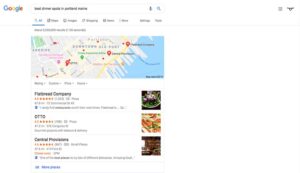This image is a blurred screenshot of a Google search results page. The background is primarily white, featuring the recognizable multicolored Google logo in the upper left corner. Directly below the logo, there is a search bar containing black text that is too blurry to decipher. Beneath the search bar are navigation tabs labeled "All," "Images," "Maps," among others. The central section of the image displays a colored map with three location pins, though the specific area is indiscernible. Directly under the map, there are review excerpts for three establishments, likely restaurants, with their names listed in black text on the left. Each establishment also shows a star rating in yellow and a color photograph positioned on the right. Lower down, there are repetitive, indistinct search bars. Three such search bars are present, but the text within them remains unreadable due to the overall lack of focus in the image.